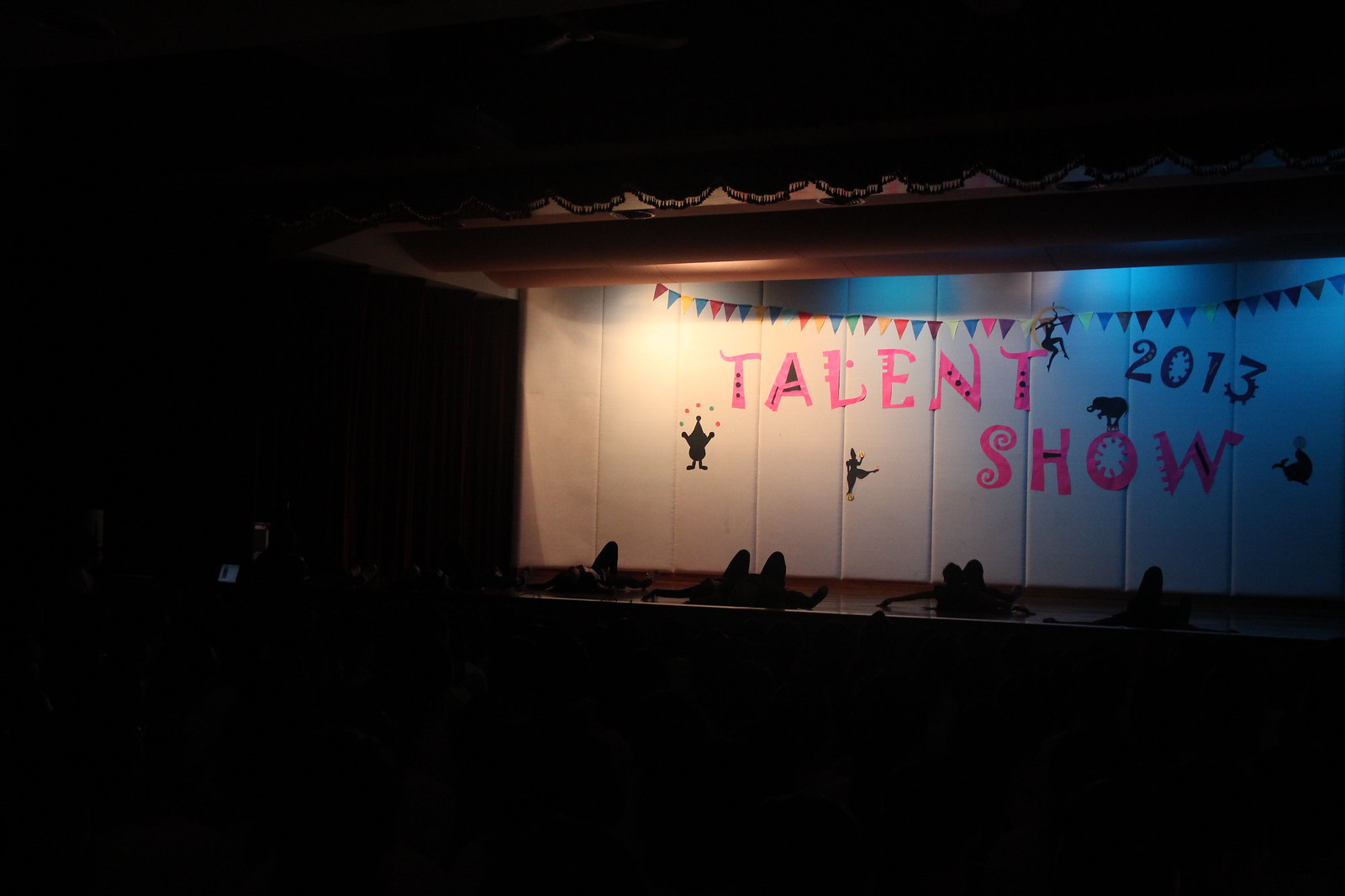The image depicts a stage set against a white-paneled wall, possibly outdoors or indoors with low lighting, creating a shadowy appearance. A colorful triangular pennant banner in shades of red, blue, yellow, orange, green, pink, purple, and black hangs across the top. Prominently displayed on the wall in vibrant pink letters is the phrase "Talent Show," with "2013" written in black above it. Adorning the wall are several black figurines; one appears to be juggling, another dancing, a third looks like a person sitting on the edge, and others might resemble acrobats or performers, adding a whimsical touch to the scene. On the lower part of the stage, partially visible under the dense shadows, are indistinct objects that seem like stacked shoes. Blue lights from the right side cast a soft hue onto the wall, enhancing the mysterious atmosphere of the setting.